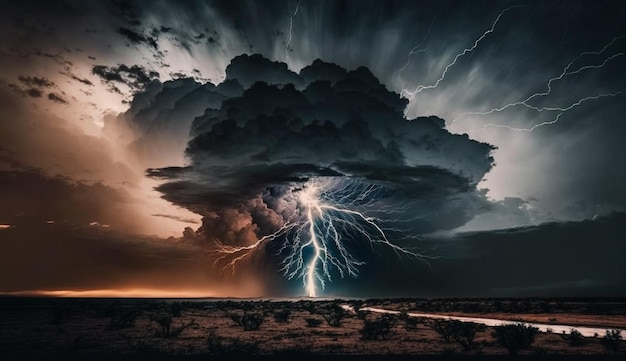This color photograph, likely a professionally done and possibly AI-generated image in landscape format, captures an intense desert lightning storm. Dominating the scene is a humongous, ominous thundercloud that occupies nearly three-quarters of the image, complete with numerous branches of lightning radiating from it. The photograph appears to be a long-exposure shot, capturing the storm in its full, eerie splendor, with one massive bolt striking the barren road below and illuminating the scene. The stark contrast of the ominous reds, greens, grays, and blacks of the cloud against the desolate, mostly brown landscape below heightens the dramatic, almost cataclysmic atmosphere. Sparse desert shrubs and bushes dot the arid ground, and a river snakes its way through the lower right corner, adding a touch of movement to the otherwise still, barren landscape. The storm cloud, thick and menacing, looks as if it’s about to engulf everything in its path, lending the scene an unsettling sense of imminent upheaval.